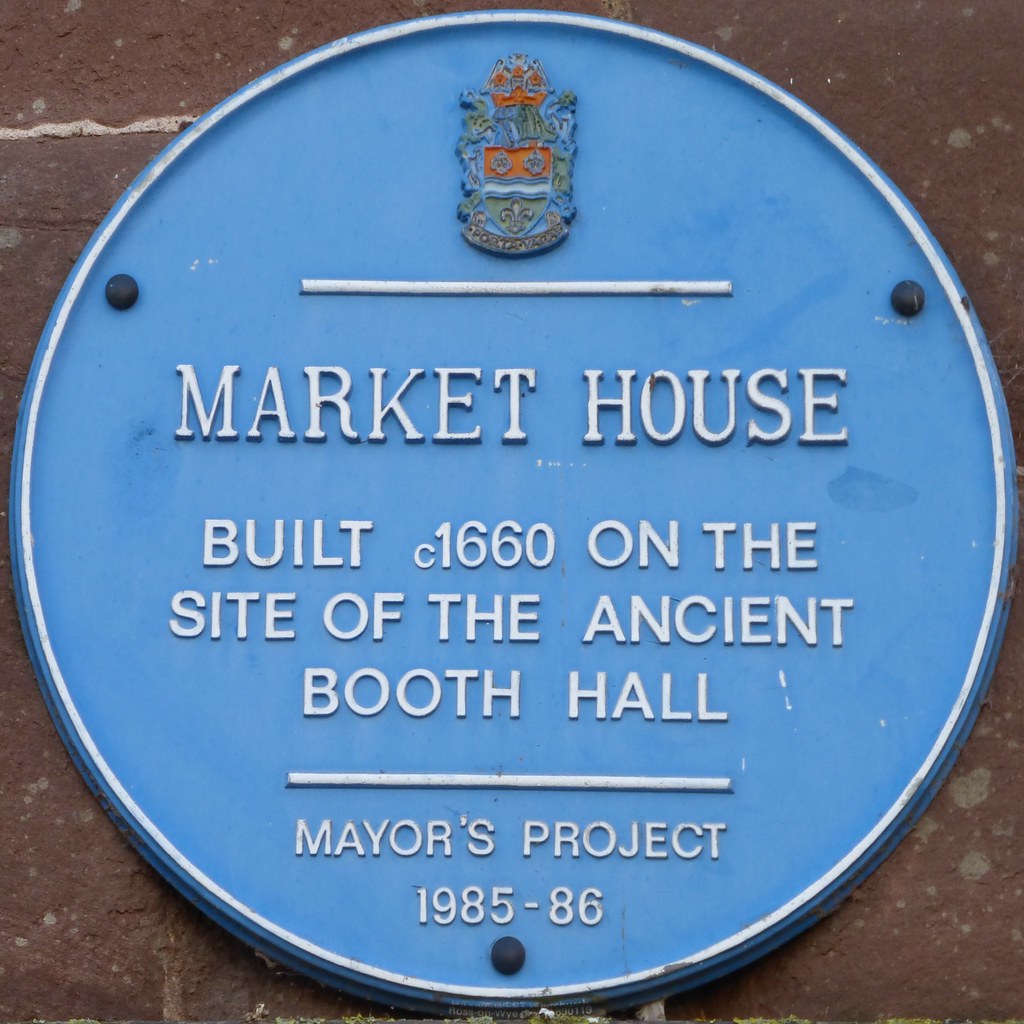This image shows a close-up of a circular memorial plaque attached to a reddish-brown stone wall, secured with three black nails. The plaque, made of painted metal, has a light blue background with a white border and features a British family crest at the top in colors including red, blue, yellow, and possibly green. Below the crest, there is a white horizontal line running from left to right. The inscription in white capital letters reads "Market House," followed by "Built c. 1660 on the site of the ancient Booth Hall" in slightly smaller capital letters. Further down, after another white line, the text indicates "Mayor's Project 1985-86" in smaller lettering.